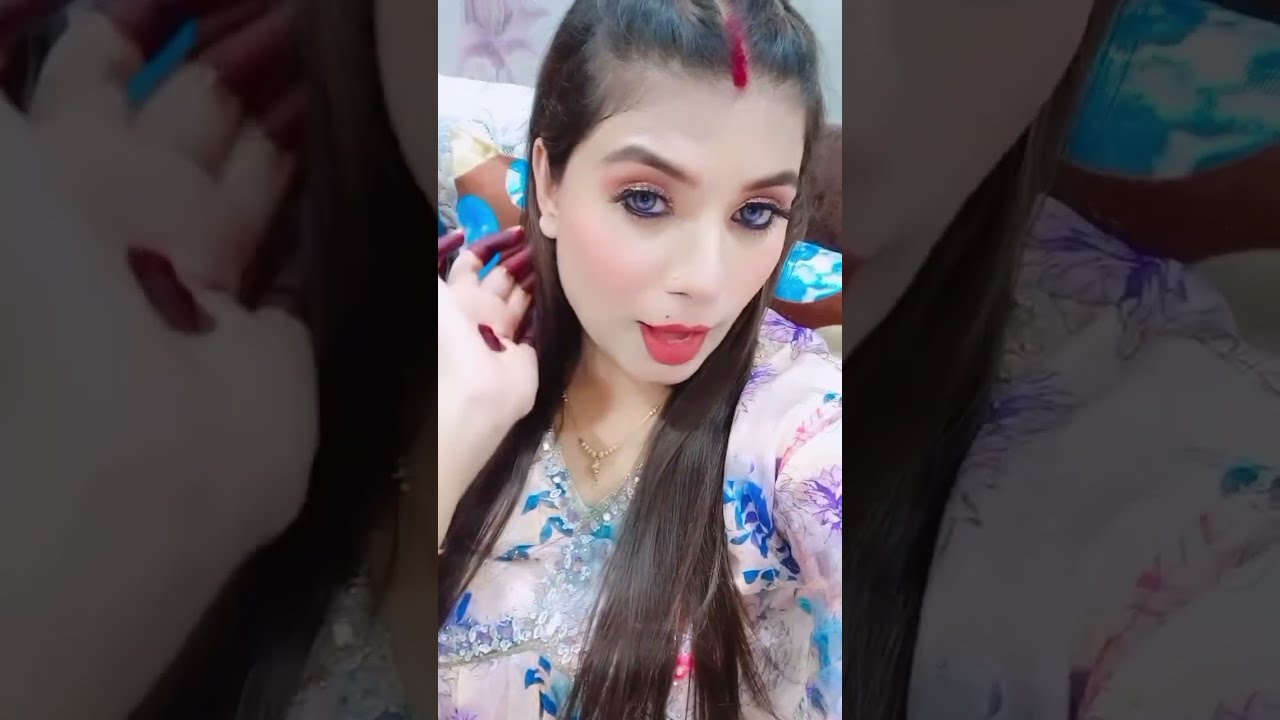The image is a detailed color photograph of a young woman with light skin and striking features, displayed in a creative collage format. At the center is a portrait of the woman with a darker filter overlay, flanked by enlarged and cropped segments of the same image. She has long, dark brown hair adorned with a distinct red streak along her center part and her fingertips are stained with dark red henna. 

The woman is wearing light brown eyeshadow, black eyeliner, long eyelashes, and possibly blue contacts, contributing to her dramatic look. Complementing her makeup, she wears deep red lipstick and has a nose piercing. Her right hand is gracefully positioned as if tucking her hair behind her ear while also revealing a red dot on her palm, emblematic of her cultural adornments. 

Her ornate outfit consists of a white silk top with blue and purple floral patterns, embellished with sequins and crystals. This attire is further accessorized with a gold-colored necklace. The background suggests a cozy, possibly pink-hued bedroom setup with colorful pillows, enhancing the overall intimate and personal aesthetic of a social media selfie. The woman’s slightly parted lips give the impression she might be speaking, adding a dynamic and lively element to the photograph.